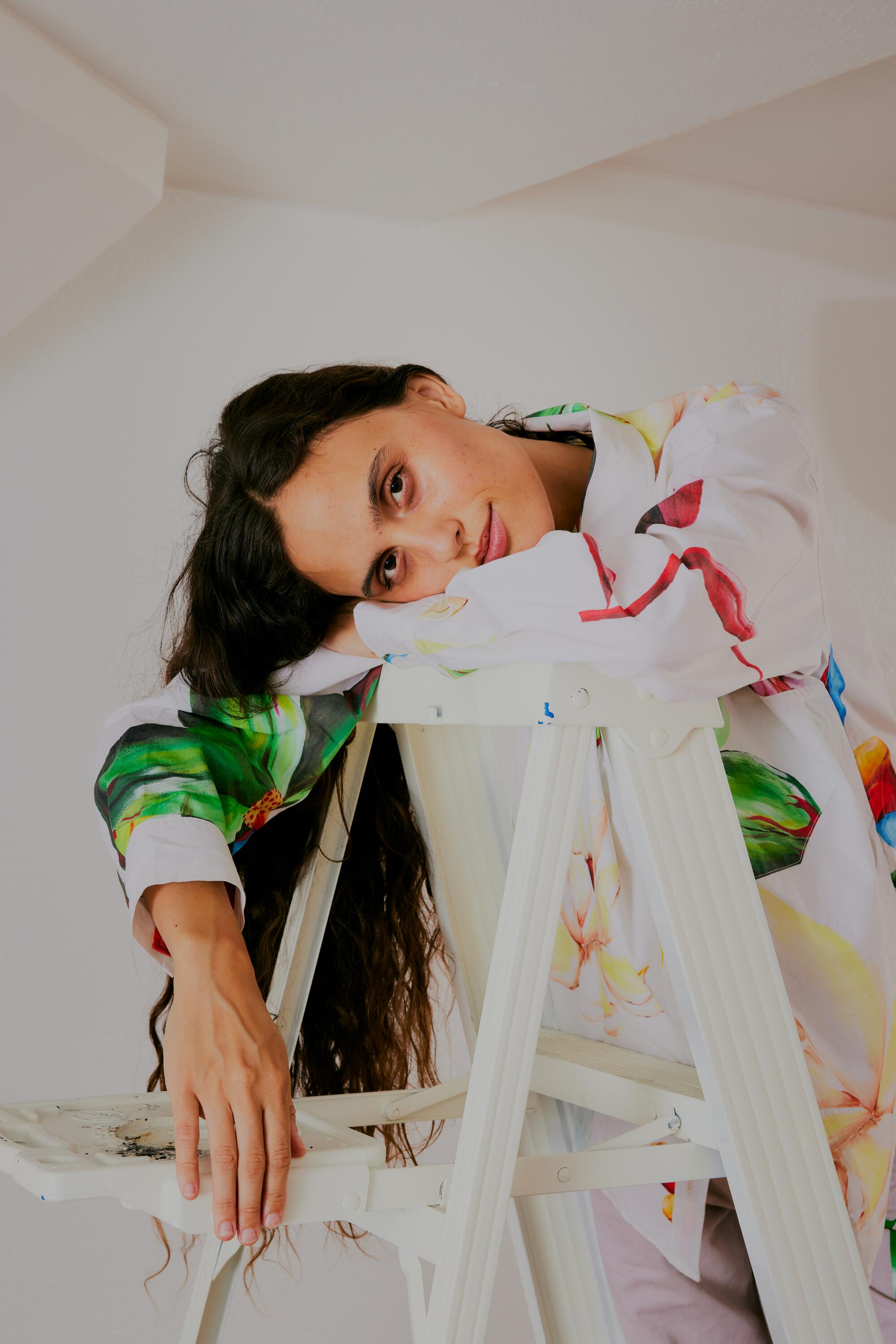This photograph is a striking portrait featuring a woman in a minimalistic, all-white room. She is leaning against a white painted ladder, her right arm resting on the top rung while her head is gently laid on her bent left arm, causing her long, dark brown hair to cascade down the ladder. She is looking straight ahead with a serene expression. The woman's outfit is particularly eye-catching: a white long-sleeve shirt adorned with vibrant watercolor patterns in pink, green, and yellow, paired with pinkish pants. The overall composition, with its contrasting elements of her colorful attire against the pristine white background and ladder, creates a visually captivating and artistically rich scene.